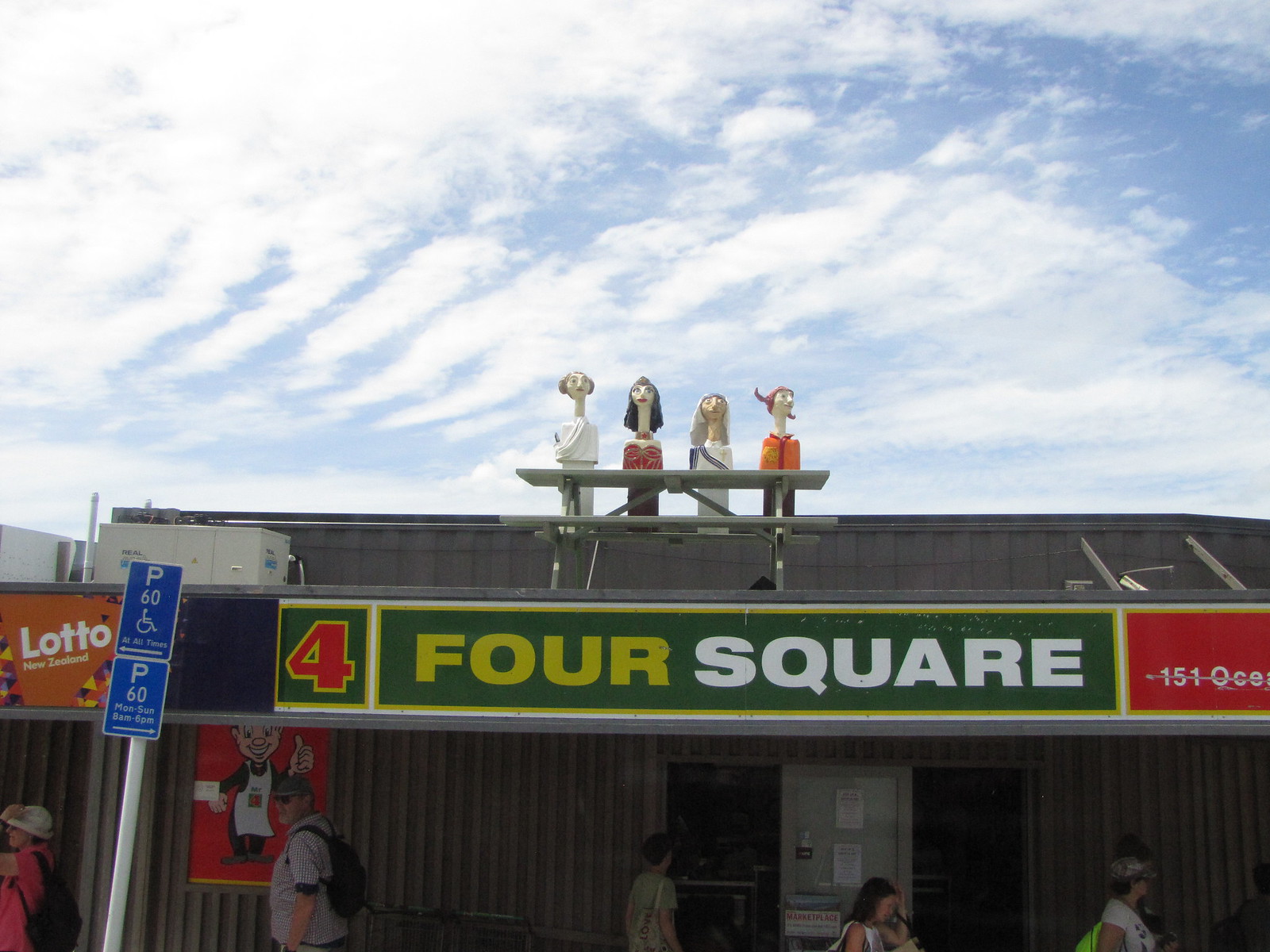The photograph features an image taken during the daytime of a single-story building, possibly a bar or shop, with a gray aluminum roof. The most striking feature is a small decorative picnic table situated on the roof, adorned with four figurines. These figurines appear to be sculpted from clay, each distinct in appearance—a figure in a white robe, another with dark black hair in a red dress, one with a gray cloth over their head and a white robe, and another with orange hair and an orange top. The table and figurines add a whimsical touch to the scene.

Below this rooftop setup, a large green sign reads "Four Square," with the numeral '4' in red bordered by yellow, and the word 'Square' in white letters against the green background. Additional text includes “Lotto” on the left and "1510CE" on the right, alongside a blue handicapped parking sign. 

In the foreground, various people of different ages and genders are seen walking past the building, although only the upper halves of the figures are visible. There’s also a small open door at the bottom. The scene is lit by daylight and the sky above is partly cloudy, with white clouds contrasting against a blue backdrop.